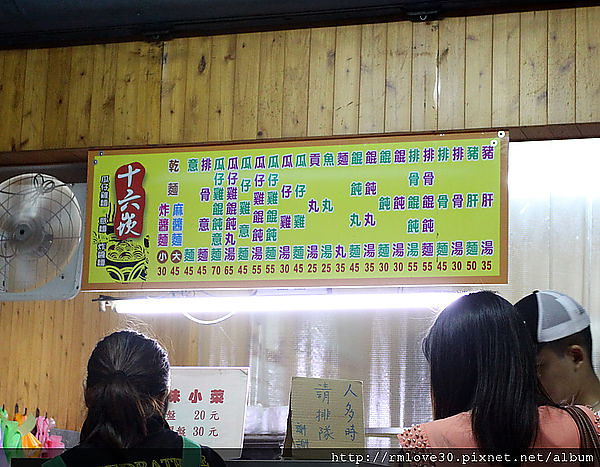In this photograph, we observe three individuals standing in front of a counter, seemingly ordering food at a restaurant in China. The focal point above the counter is a vibrant yellow, purple, and green sign adorned with Chinese characters which likely serves as a menu. This sign includes numbers ranging from 30 to 70, possibly indicating prices. To the left of the sign, a fan is mounted on the wood-paneled wall, which extends horizontally across the establishment. The individuals' backs are to the camera, with the man on the right wearing a baseball cap, a woman in pink with medium-length black hair standing next to him, and another woman with long, dark hair tied in a ponytail on the left. Additionally, there are two smaller signs with characters and numbers in front of the trio, hinting at additional menu items or prices. Lastly, a small watermark in the lower right of the image reads "http://rmlove30.pixnet.net.album."